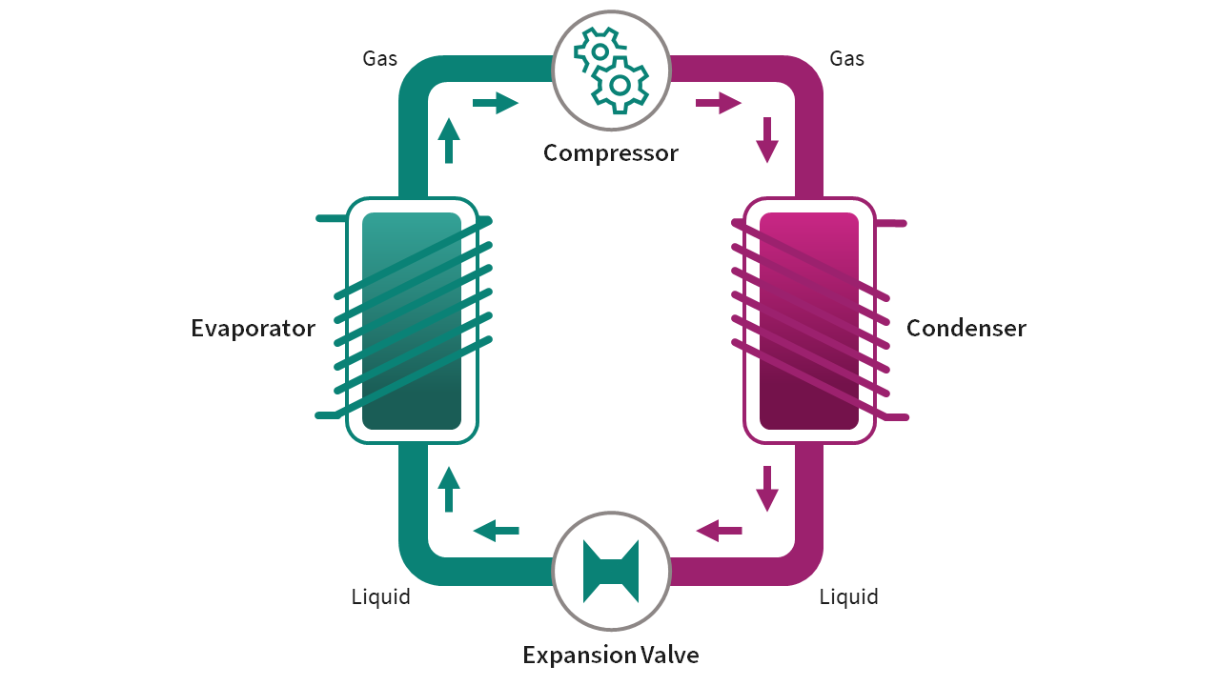The image is a detailed drawing of a flow chart on a white background, prominently featuring both green and deep pink (magenta) colors. The diagram, which is rectangular with long vertical sides, outlines an interconnected process involving several key components labeled in black text. Starting at the top center, there is a circle containing gear shapes labeled "compressor," from which a pink arrow labeled "gas" points to the right. The diagram then follows a sequence of elements outlined in magenta on the right side and green on the left.

To the top right, a rectangle resembling a cell phone, labeled "condenser," contains diagonal pink bars and is flanked by a pink arrow at the bottom marked "liquid." Another pink arrow leads downward to a circle at the bottom center, containing a symbol akin to a bow tie or a spool, labeled "expansion valve." Transitioning from here, a green arrow labeled "liquid" points to the left.

Further up on the left side, a green rectangle labeled "evaporator" mirrors the cell phone shape and is again marked by diagonal lines, this time in green. A green arrow labeled "gas" ascends from this evaporator back towards the initial compressor, completing the cyclic flow.

Throughout the diagram, arrows guide the viewer through the described process, highlighting the transformation from gas to liquid and back to gas, indicative of an evaporation cycle. The use of directional arrows throughout the corners and sides of the image emphasizes the cyclical nature of the process depicted.